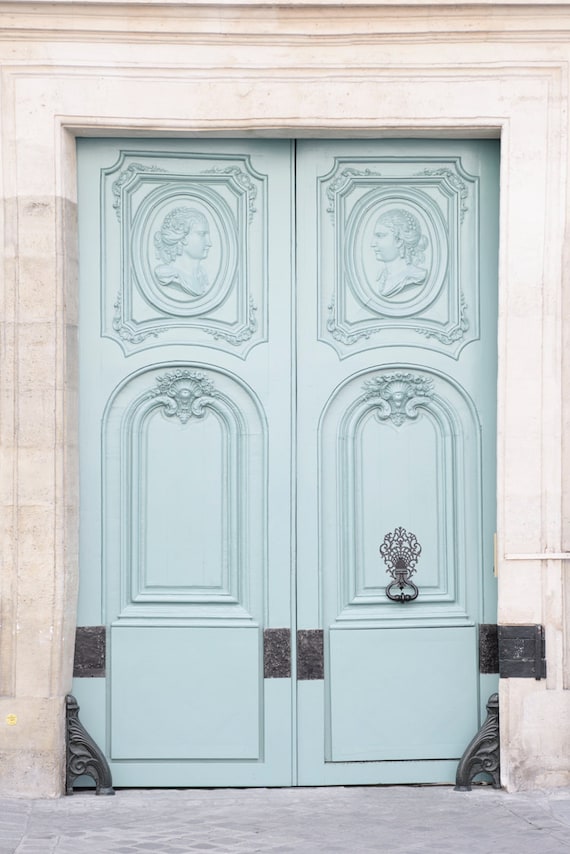The image focuses on a pair of ornate, photorealistic, double front doors centered in the frame, extending nearly to the edges and top and bottom of the shot. These doors are a light, greenish-blue color and exhibit intricate detailing. Most prominently, at the top of each door is a finely carved bust of a noble or royal lady in profile, her hair elegantly styled, evoking a sense of vintage art.

The right door features a black metal knocker positioned around three-quarters of the way down. Both doors are adorned with dark rectangular insets, strategically placed towards the edges: one near the middle, another at the opposing edge, and two near the hinges, enhancing the decorative motif. At the base of each door, ornate elements extend into the building’s structure, serving both decorative and functional purposes.

The surrounding door frame is made of ornate white stone or marble-like material, complementing the doors' intricate designs. The ground outside the entrance is paved with gray tiles, maintaining the overall refined aesthetic. The photograph captures the door in a minimalistic setting, stressing its sophisticated and vintage-inspired design without any visual clutter.